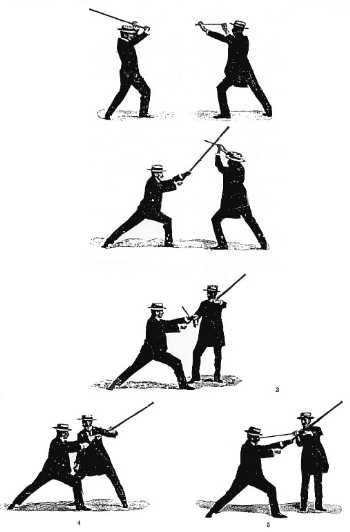This black-and-white image series, rendered in different shades of grey, depicts five sequential illustrations reminiscent of an old dueling manual or cinematic fight scene. Two well-dressed men, clad in black suits and bowler hats, are engaged in a sword-fighting or stick-fighting sequence. In the topmost illustration, both men raise their sticks, poised to strike; one holds his stick defensively with both hands. The second illustration captures the clash, with the man on the left striking and the one on the right blocking the blow. In the third scene, the attacker shifts his angle of assault, while in the fourth, his attack is parried. By the fifth and final image, the defender has countered with a face-targeted strike. The evolution of their duel is shown step-by-step in a progressive, narrative style, immersing the viewer in the dynamics of the fight.